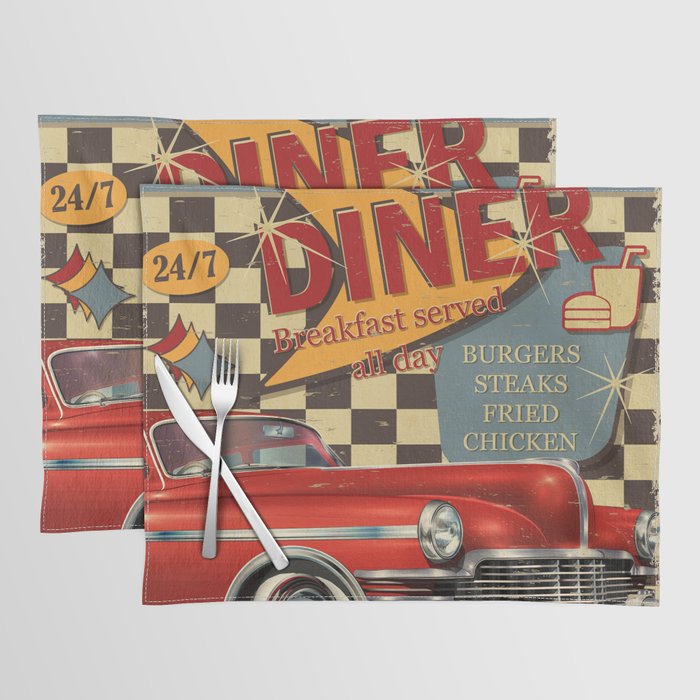The image depicts two offset cloth placemats adorned with a vibrant 1950s diner-themed design. Each placemat showcases an old-fashioned diner menu atop a black and white checkered background. Dominating the top left corner, a yellow oval boldly announces "24-7." To the right, a large yellow boomerang shape with a black outline frames the word "DINER" in prominent bold letters, each adorned with white stars. Below, the menu proudly declares in red lettering, "BREAKFAST SERVED ALL DAY." The placemats feature a semi-rectangular blue section listing "BURGERS, STEAKS, FRIED CHICKEN" with accompanying simple cartoon icons of a burger and a drink with a straw. The lower section prominently displays an old-fashioned red car with silver trim and headlights. Cartoon images of a crossed fork and knife sit atop the car, adding to the retro feel. Additionally, the far left side features a trio of overlapping diamonds in red, yellow, and blue, forming a striking background for the utensils.